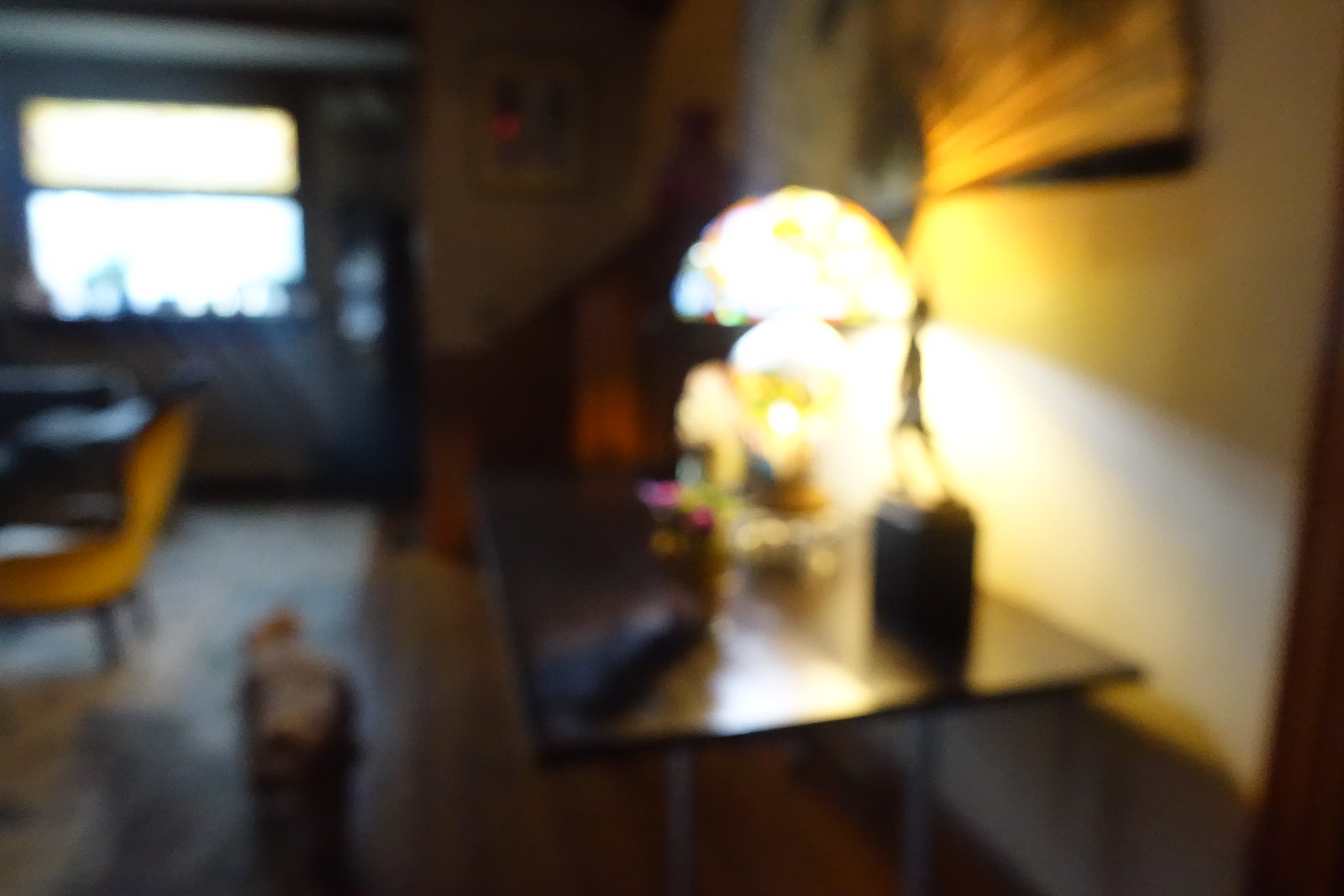The photograph depicts a mostly out-of-focus indoor scene with a brown wooden floor stretching across the frame. On the left side of the image, a glimpse of the sea can be spotted, merging seamlessly with the backdrop. In the distant background, a light source is faintly visible, casting a mild illumination throughout the room. The right side of the photograph features a white wall adorned with a few mounted fans. A lit lamp further brightens this section, standing out amidst the otherwise blurred surroundings. In closer focus within the scene, there appears to be a statue positioned on a black base, with a person standing beside or on it. In the forefront of the image, the edge of a brown wooden tabletop slightly emerges, though its finer details remain indistinct due to the overall lack of clarity.